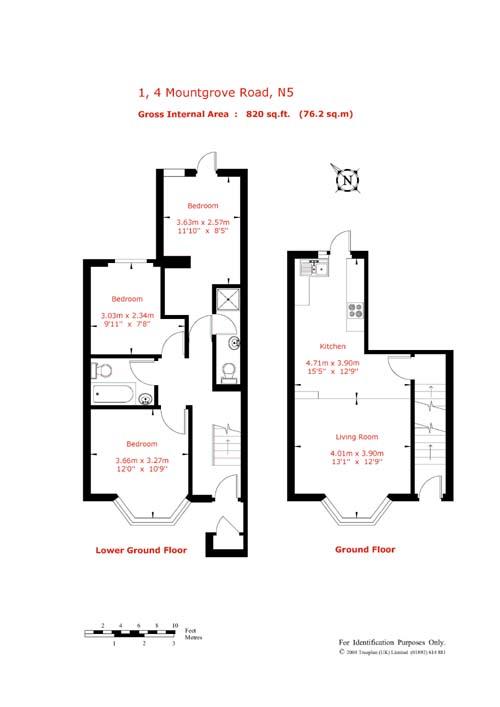This image features a detailed architectural blueprint for a house located at 1-4 Mt. Grove Road, N-5. At the top of the blueprint, highlighted in red text, the gross internal area is specified as 820 square feet or 76.2 square meters. Below this information, a compass symbol is displayed, with an "N" and an arrow pointing diagonally to the upper left, indicating the direction of north. 

The main section of the blueprint is divided into two parts. On the left side, labeled in red at the bottom, is the "Lower Ground Floor." This portion of the blueprint, outlined in black, illustrates a layout of six distinct rooms, each containing small, red inscriptions that are unreadable due to the insufficient clarity when zoomed in. 

On the right side, marked in red as the "Ground Floor," the blueprint similarly outlines three rooms, each containing small red text. Below these blueprints, there is an additional section of writing that remains unreadable in the image. Additionally, to the left of this section, there is a black and white line with inscriptions positioned above and beside it, which are not decipherable in the current resolution.